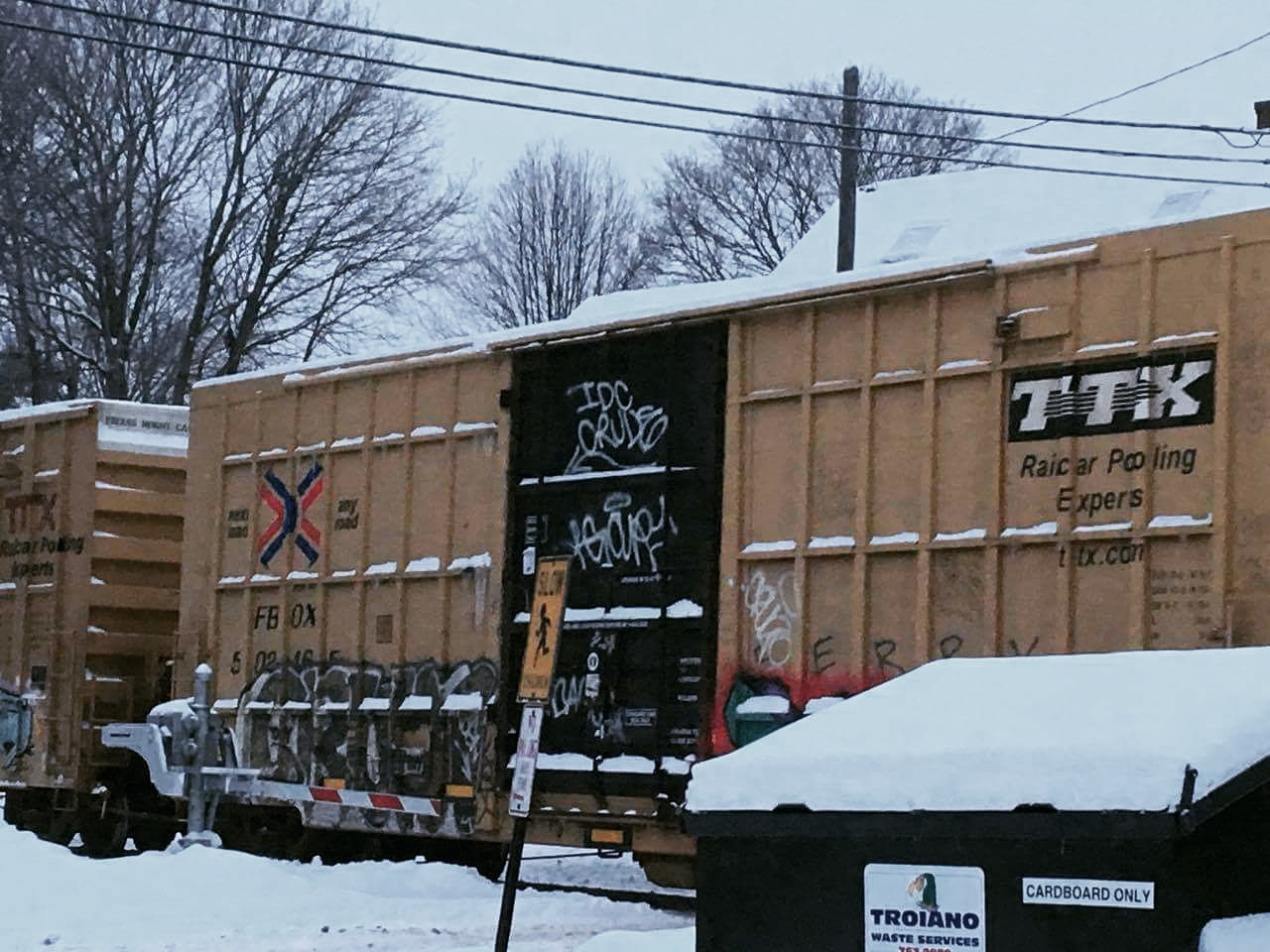This outdoor winter scene features a hazy, overcast sky with thin, leafless trees fanning out, their barren branches creating a dense, intricate pattern against the white backdrop. Dominating the mid-ground are several tall, brown cargo train containers adorned with tan labeling stating "TTX Railcar Pooling Experts," with one of the containers displaying graffiti on its closed black door. These railcars, with snow delicately dusting their tops and some ribbing, are arranged on tracks that lead from the lower left-hand side to the center-right side of the image. In the foreground to the right, there is a darker brown dumpster also covered in snow, prominently labeled "Triano Waste Services" and designated for cardboard recycling. Additional details include a partially visible building with a snow-covered roof behind the railcars and three power lines extending from a pole, contributing to the industrial ambiance. Snow blankets the entire ground, enhancing the cold, wintry atmosphere of the setting.